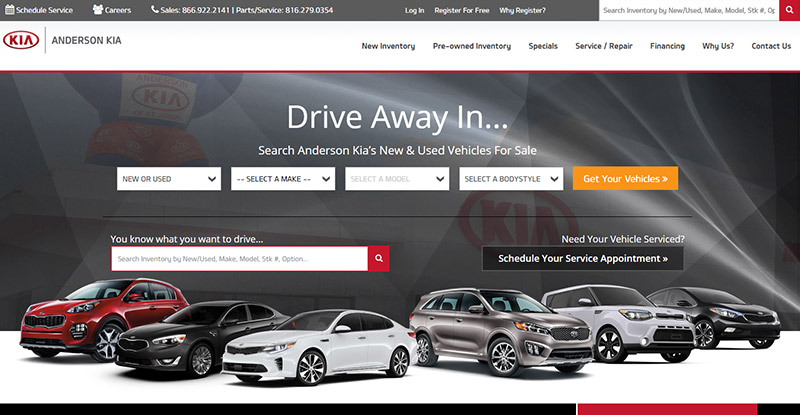Screenshot of the Kia Automobile Website's Homepage

The screenshot captures the homepage of the Kia automobile website, likely viewed on a laptop or desktop. The top left corner features a gray rectangular box extending three-quarters of the way to the right. Inside this box are several icons:
- A clipboard icon labeled "Schedule Service"
- An icon of people labeled "Careers"
- A phone cradle icon labeled "Sales: 866-922-2141"
- An icon resembling an "i" (information) labeled "Parts Service: 816-279-0354"
- The words "Login" in white lettering
- The phrase "Register for Free"
- The question "Why Register?"

Next to these icons, there is a white search bar labeled "Search inventory of new/used make model, make model, STK, or STK number". To the immediate right is a red box with a white magnifying glass icon.

In the upper left corner of the page is a red oval with white lettering "KIA" flanked by a gray vertical line and next to it, "ANDERSON KIA" in all caps. Extending right from this area are navigation links: "New Inventory", "Pre-Owned Inventory", "Special Service/Repair", "Financing", "Why Us?", and "Contact Us", all in gray lettering on a horizontal line.

Below this navigation bar is a thin horizontal red border sitting above a dark gray background embossed with faint Kia logos and designs. The main headline in the top-middle area reads "Drive away in…" in large letters, followed by smaller white text stating, "Search Anderson Kia's new and used vehicles for sale".

Directly below this headline are five rectangular search bars:
1. White background "New or Used" with a downward arrow
2. Gray text "Select a Make" with two dots and a downward arrow
3. Light text "Select a Model" with a downward arrow
4. "Select a Body Style" with a downward arrow
5. An orange background button labeled "Get Your Vehicles" with an arrow pointing right

Beneath these search bars, a thin black horizontal line emphasizes the search section. Below this, a red-bordered search box provides options to "Search inventory by new/used, make model, STK number". Next to this is a black box with white text, posing the question: "Need your vehicle serviced?", and below it, a button labeled "Schedule Your Service Appointment" with arrows pointing right.

Further down, images of various Kia cars appear angled across the screen in different colors including red, black, white, and silver, facing either left or right. Lastly, near the bottom of the screenshot is a horizontal bar, transitioning from black to a small white vertical line, a red section, and back to black.